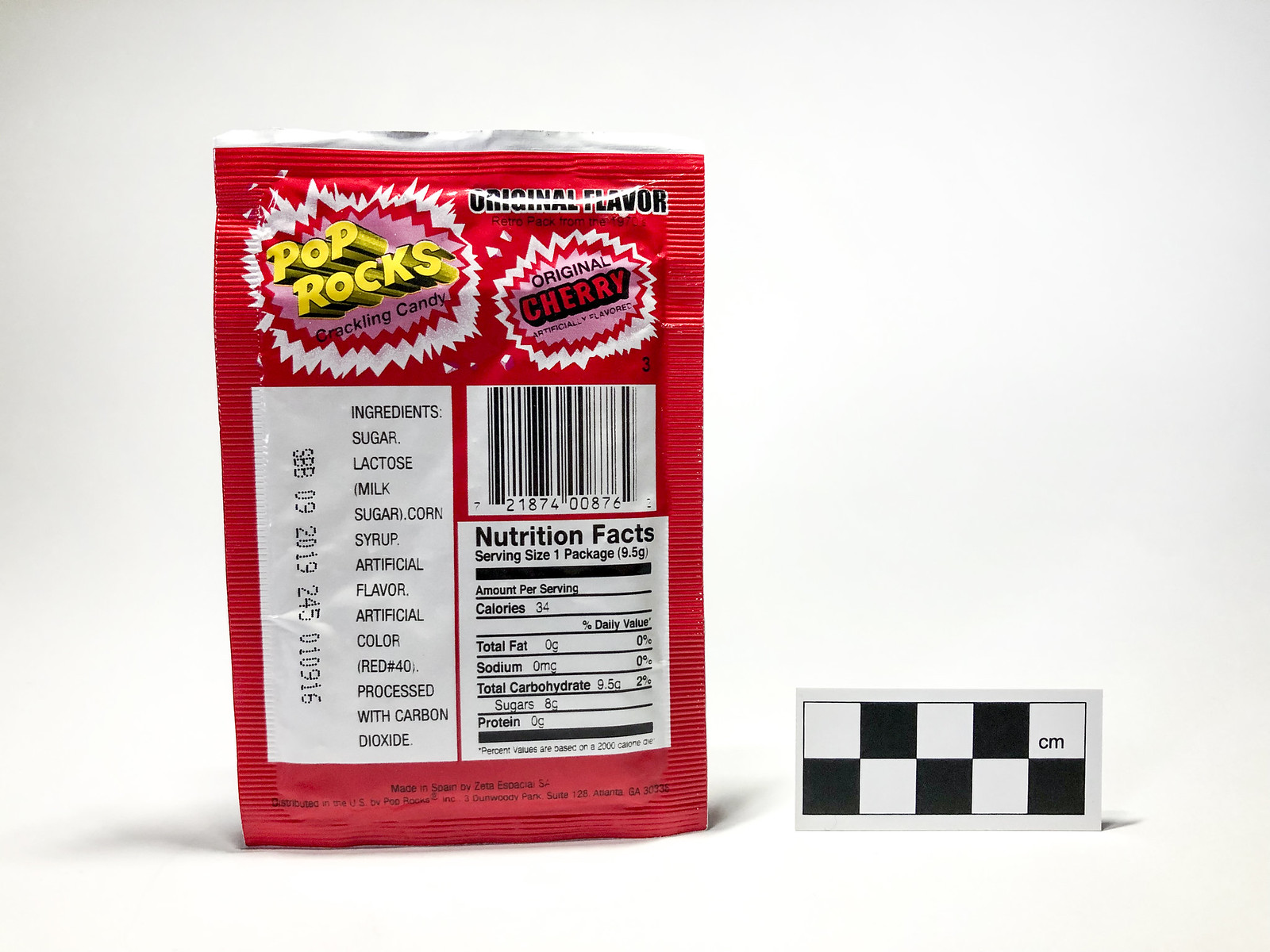This image features a bag of Pop Rocks and a rectangular piece of cardboard with a black and white checkerboard design. The cardboard has five columns and two rows arranged in a checkerboard pattern on a white background, with the word "centimeters" printed between the right and left blocks, resembling a ruler.

The Pop Rocks candy bag is shown from the back, revealing the ingredients list, production time, and lot number, indicating that it was made in September 2019. A white square in the lower right corner displays the Nutrition Facts, and a barcode is located above this section. At the top of the bag, the words "Original Flavor" are printed. The packaging features a lively design with starburst shapes in white, red, and pink. The left side of the packaging prominently displays the brand name "Pop Rocks" in yellow, along with the description "Crackling Candy." On the right side, in a smaller font, it reads "Original Cherry" with a note that it is artificially flavored.